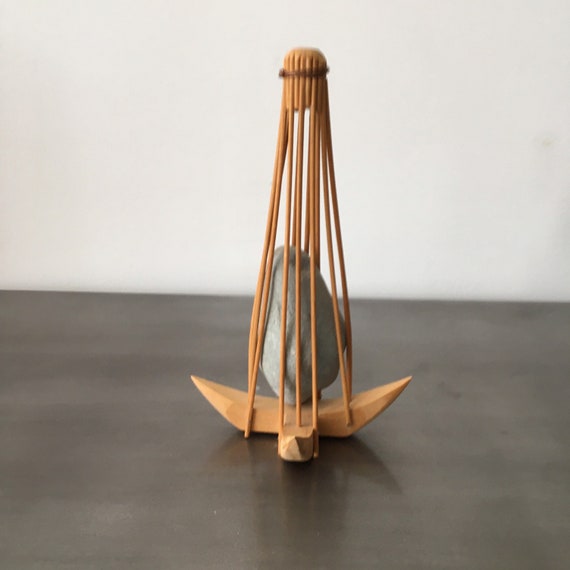In this image, we see a decorative object positioned on a dark brown, almost black table with a distinct white background. The object itself is a light gray stone of an irregular, oblong shape, resembling a piece of clay or rock, and resting upright. Enclosing the stone is a cage-like wooden structure featuring slender, pointed legs; these legs protrude from each side of a wooden base, totaling four legs altogether, though only three are visible from this angle. This wooden structure, brownish in hue, tapers towards the top, creating a shape reminiscent of an upside-down diffuser or a wine cork. The reeds or bars form a narrow enclosure around the stone, conferring a sense of the stone being encased or jailed. The overall color scheme of the image is quite monotone, featuring shades of white, gray, black, and varying browns, adding to the minimalistic aesthetic of the scene.